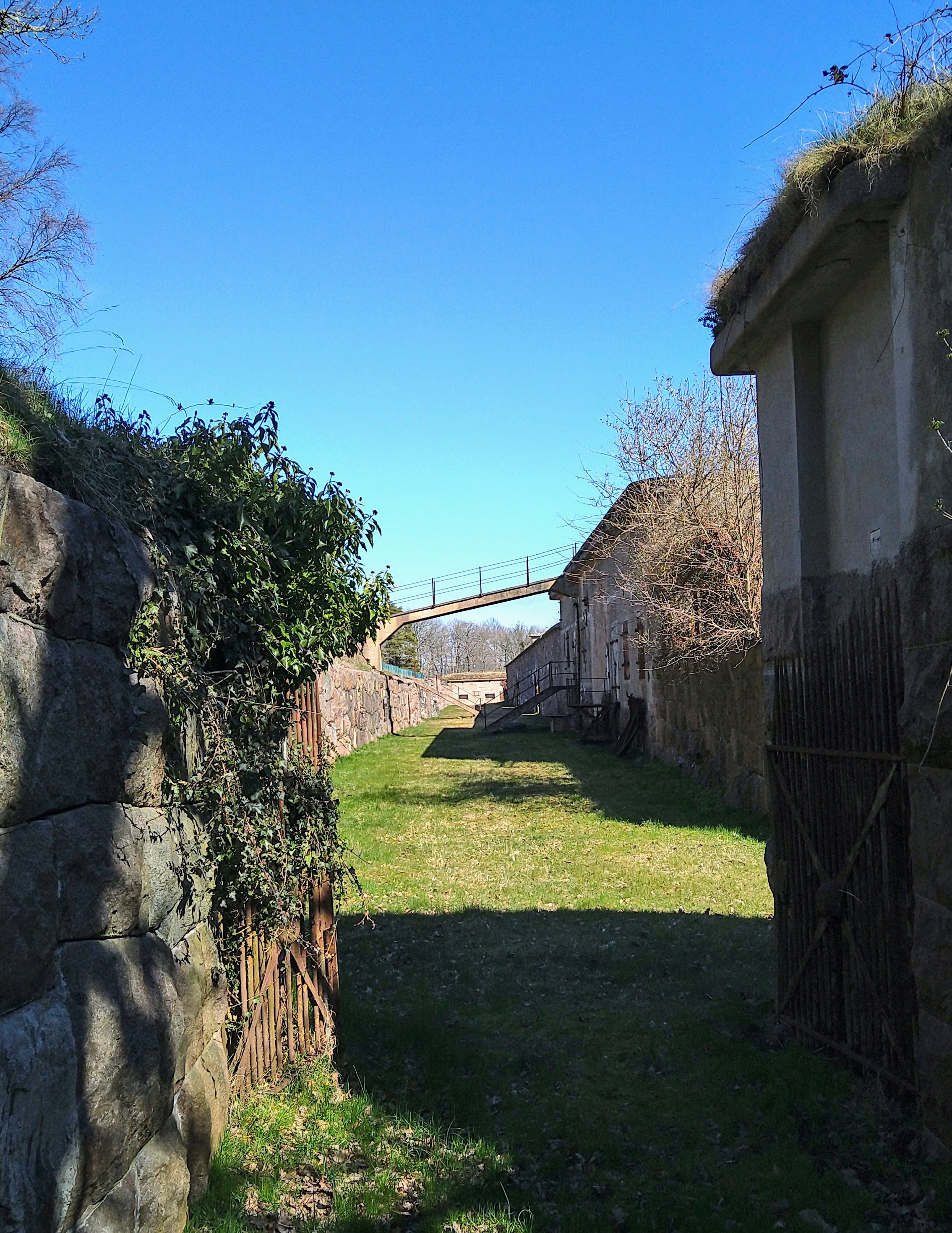The photograph captures a scene of a country property characterized by a bright blue sky overhead. In the foreground, a vibrant green lawn is divided into areas of heavy shadows and sunlit patches, suggesting sunlight streaming from an unseen source. Prominently featured on the left side of the image is a substantial stone wall, while to the right, a collection of older beige buildings, possibly stucco or stone, bordered with vines and random plants like ivy, forms a rustic backdrop. There is a notable black gate that stands out amidst these structures. The middle ground reveals a narrow expanse of grass separating the stone wall and buildings, implying a shared backyard space among multiple residences, devoid of fences. Towards the background, a slanted structure, possibly a train bridge or walkway, extends down to the fence line. The top part of the image showcases a tree on the left and a white building further in the distance, contributing to the rural ambiance of the scene.